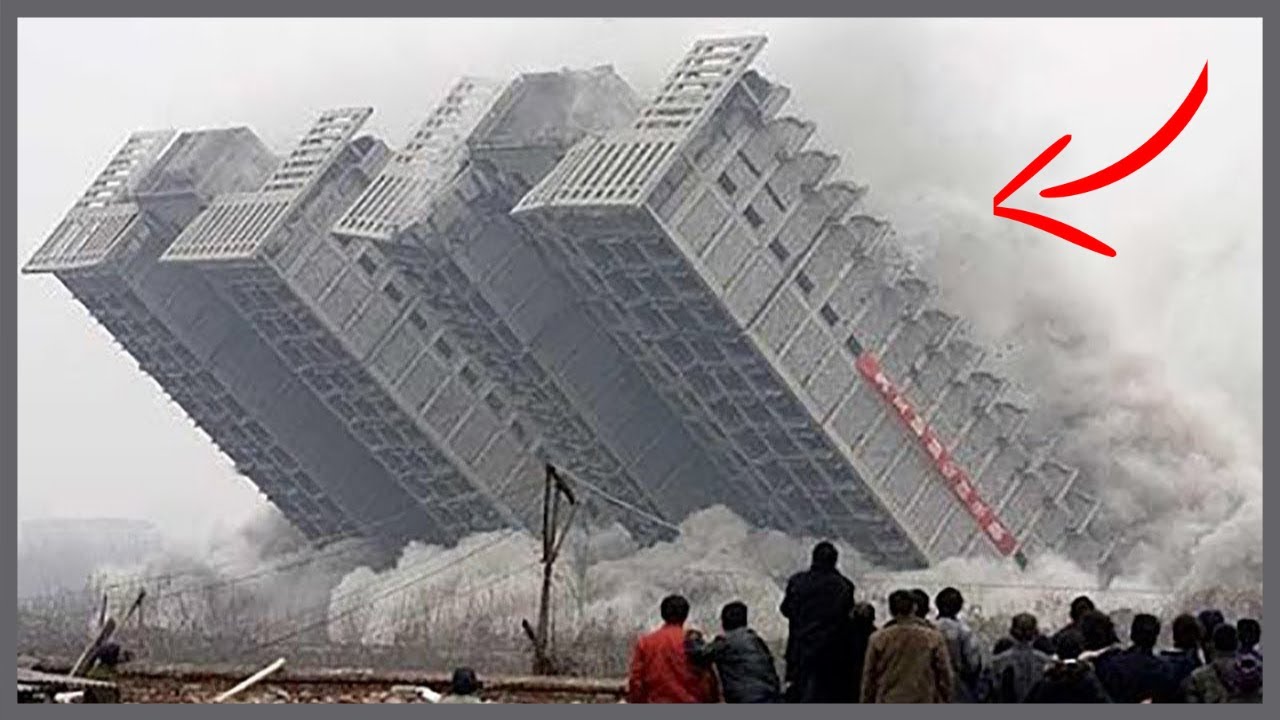The horizontally aligned rectangular picture, framed by a dark gray border, captures the dramatic demolition of four tall, vertical, rectangular buildings. These gray buildings, each around 25 to 30 stories high, tilt at approximately 45 degrees as they collapse simultaneously amid a cloud of smoke and dust. The building closest to the right boasts a distinctive vertical red sign with white symbols, indicative that the scene is set outside of the United States. An added red arrow in the upper right corner points to this uniquely marked building. In the lower portion of the image, a group of spectators stands about 500 yards away, observing the event from a safe distance, with a few telephone poles visible in the foreground.